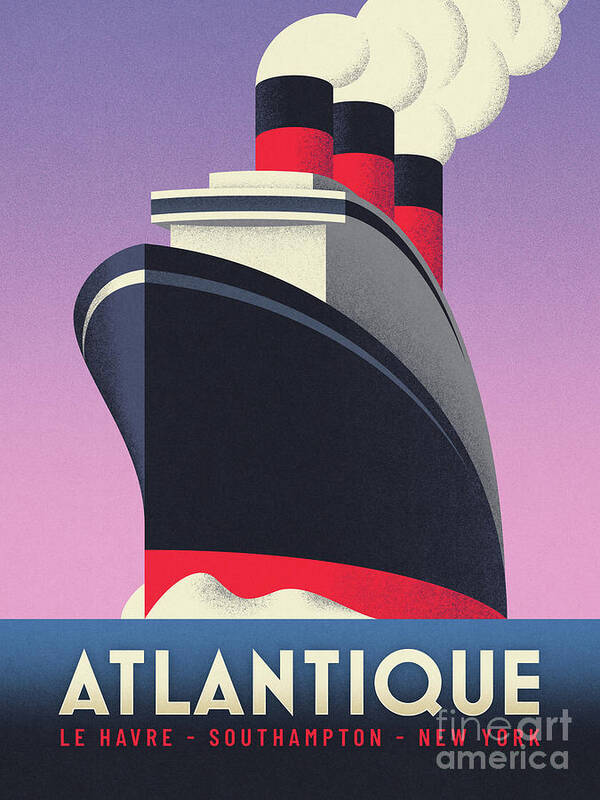This image is an Art Deco style poster that resembles a classic postcard or postage stamp, featuring a striking depiction of an ocean liner. The ship is illustrated with elegant precision, showing a red keel and a black hull with a white strip running across the middle. Above the hull, the superstructure is white, and the ship boasts three prominent steam stacks, each red at the base and black at the top, emitting white smoke. The vessel is portrayed in dynamic motion, as evidenced by the white wake at its base, giving the impression of it sailing forward out of the poster.

The background showcases a gradient starting with a purplish hue at the bottom that transitions into a darker, bluish-purple at the top. At the very bottom of the image, a blue rectangular border contains white text that reads "Atlantique," with the ports of call listed beneath as "Le Havre - Southampton - New York." A watermark in the bottom right corner states "Fine Art America," subtly blending into the overall design. The poster, with its vivid colors and streamlined design, captures the nostalgia and grandeur of early 20th-century passenger liners.